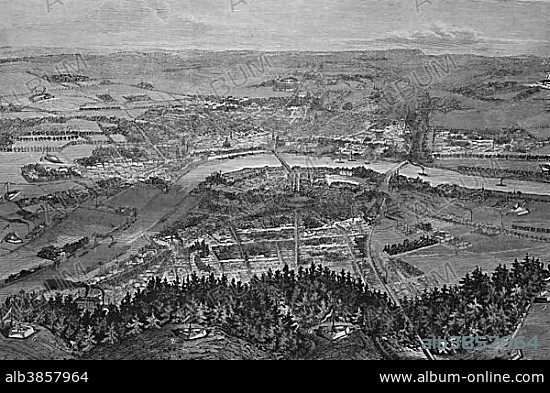This is a very old, aerial black-and-white photograph or print, likely taken many years ago, featuring the faint imprints of age and wear. Captured from a high vantage point, the panoramic image offers a sweeping view of a town etched into the landscape below. The scene prominently showcases a meandering river that elegantly snakes through the middle of the photograph, intersected by two bridges. Surrounding the river, you can delineate a wavy tree line marking the forest's edge, with darker and lighter trees adding contrast to the monochromatic palette. Beyond the forest lies an intricate patchwork of roads, plots of land, and scattered homes indicating both urban and agricultural development. Some plots remain empty, hinting at future growth. You can also notice a significant building near the riverbank and a few boats dotting the waterway. The distant background features silhouettes of mountains, adding depth to the photograph. The sky above shows some clouds, creating a dynamic conjunction between land and sky. At the bottom of the image, a black band contains the text "ALB3857964" on the left and "www.album-online.com" on the right, suggesting the photograph is part of an archival collection.